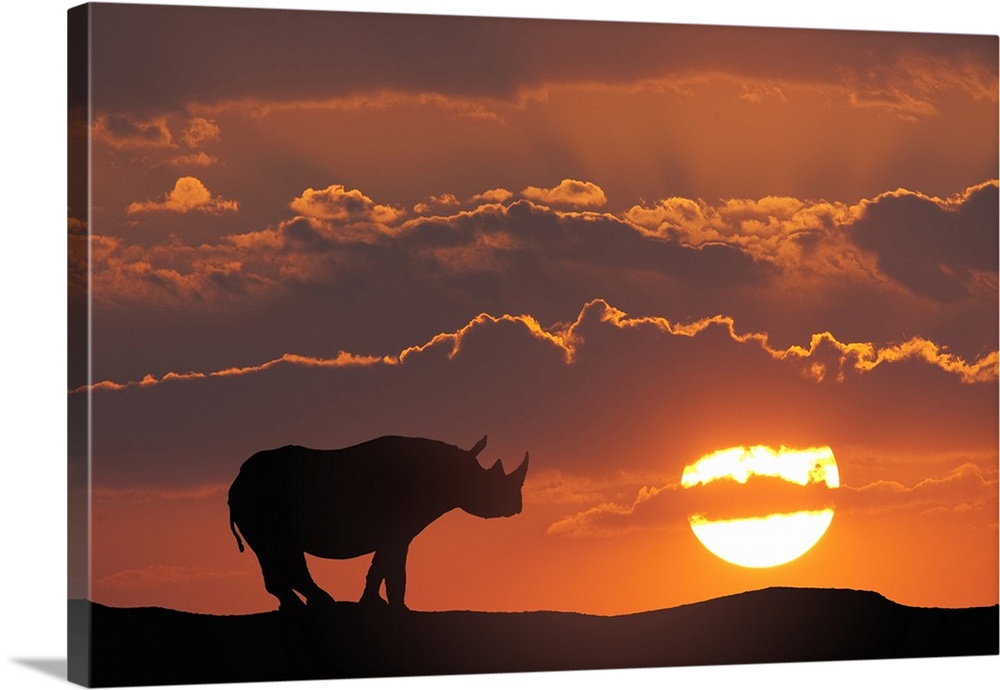In the image, a silhouette of a rhinoceros is prominently featured, standing on a nondescript piece of land, facing right. The rhino is depicted in profile, showcasing its entire form from the tip of its horn down to its tail. The background is an expansive, richly colored sky at sunset, filled with hues of deep red, brownish red, and orange. A bright, yellowish sun sits low on the horizon, partially obscured by streaks of purple-tinged clouds that are scattered across the sky in waves. This scene is not just a flat picture, but a painting on a canvas with a 3D effect, wrapping around the sides for a more immersive and tangible appearance, making it suitable for hanging as a decorative piece.